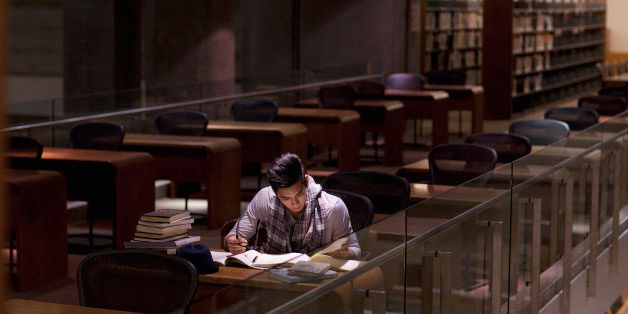The photograph, taken indoors at night, depicts a dimly lit library interior dominated by dark brown and beige tones. The image, approximately two inches high by six or seven inches wide, features blurry rows of bookshelves in the background, filled with indistinguishable books. In the foreground, a young man with dark hair and a light-colored jacket is intently studying at a curved, wooden desk illuminated by a focused light. The desk is scattered with open books and papers, with a pen in his hand and another pen resting on a page. To his left, there is a stack of additional books. Surrounding him, empty black chairs accompany other wooden desks, some facing the camera and others oriented differently. A glass rail can be seen extending along one side, adding to the structured yet shadowy ambiance of the room.